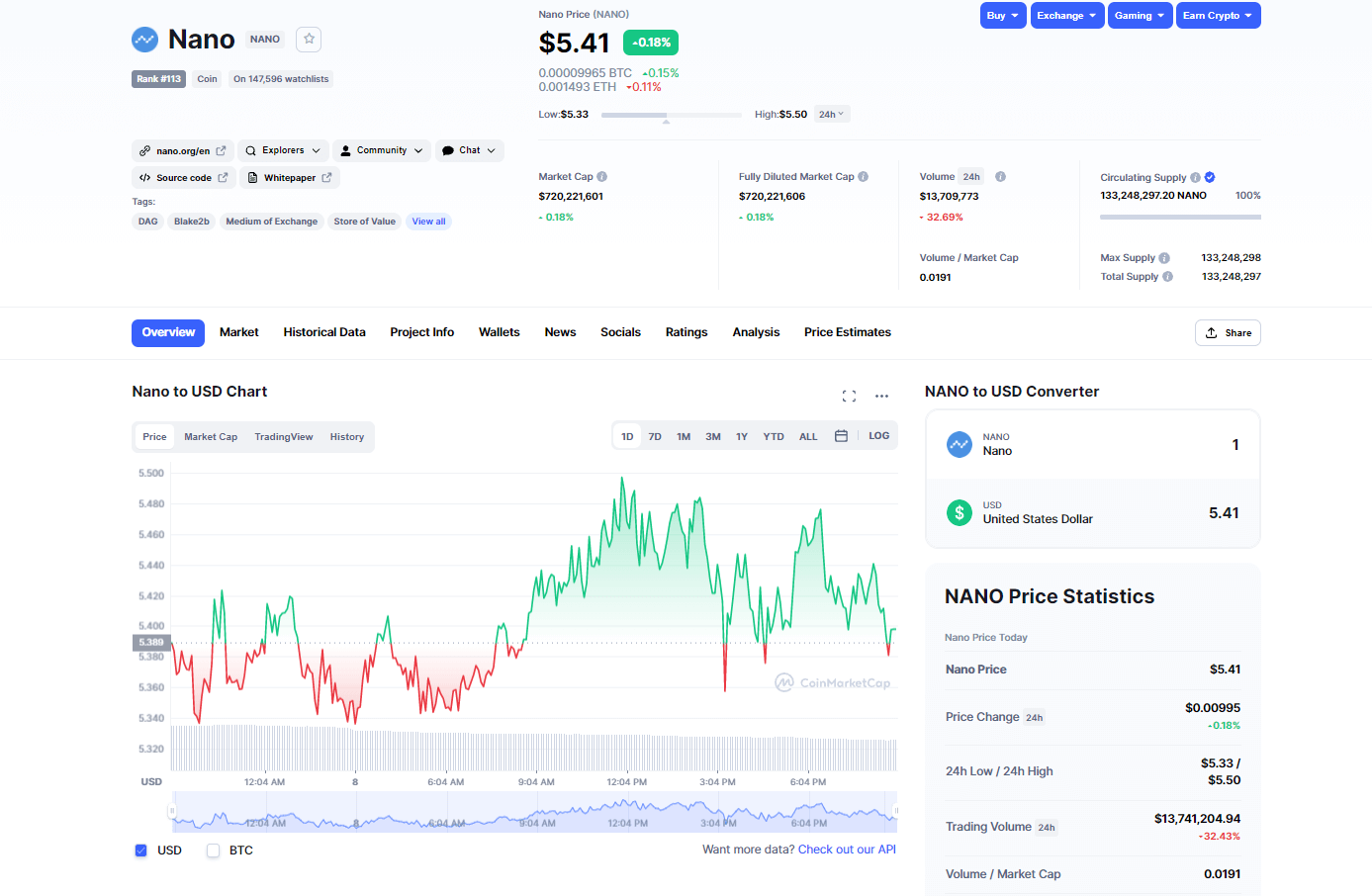The graphic presents detailed information about the cryptocurrency Nano. The top of the image features a branding section where "Nano" is written in black next to a small blue circle with a wavy white line inside. Below "Nano," the text shows the rank (#113) and mentions that this coin is on 147,596 watchlists.

The center section displays Nano's current price, which is $5.41, indicated in black text. To the right, a green banner highlights a price change of -0.18%. Further, the image provides various statistics including the price in Bitcoin (BTC) and Ethereum (ETH). Specifically, Nano has dropped -0.15% against BTC (indicated in green) and -0.11% against ETH (indicated in red). The graphic also shows a 24-hour price range with a low of $5.33 and a high of $5.50.

Several interaction buttons are positioned in the upper-right corner: "Buy," "Exchange," "Gaming," and "Earn Crypto," each within a blue banner with downward arrows indicating clickable dropdowns. On the left-hand side, navigational links to categories such as "nano.org/en," "Explorers," "Community," "Chat," "Source Code," and "White Paper" are available.

Tags associated with Nano are mentioned, including DAG, Blake 2B, "Medium of Exchange," and "Store of Value," followed by a "View All" link in blue. Further below, financial details are provided:
- Market Cap: $720,221,601 with a change of -0.18% in green.
- Fully Diluted Market Cap: Same value and percentage change as the Market Cap.
- 24-Hour Volume: $13,709,773 with a -32.69% change in red.

Additional metrics such as Volume/Market Cap, Max Supply, Total Supply, and Circulating Supply with corresponding values and percentages are listed. Above these, a share button is available.

At the bottom center, there are tabs for “Overview,” “Market,” “Historical Data,” “Project Info,” “Wallets,” “News,” “Socials,” “Ratings,” “Analysis,” and “Price Estimates,” with "Overview" highlighted in blue with white letters.

The image includes a Nano to USD price chart, colored red and green, showing price fluctuations over time. Price details range from $5.32 to $5.50, and time intervals (e.g., 12:04 AM to 6:04 PM) are displayed along the bottom. The "USD" price view is checked by default, while "BTC" is not selected. 

Finally, a prompt for more data suggests checking out their API, linked in blue. A Nano to USD converter is also available, illustrating that 1 Nano equals $5.41 USD, represented with a blue and green circle. Below, a "Nano Price Statistics" section details additional price metrics, including the current price, 24-hour price change, trading volume, and volume market cap.